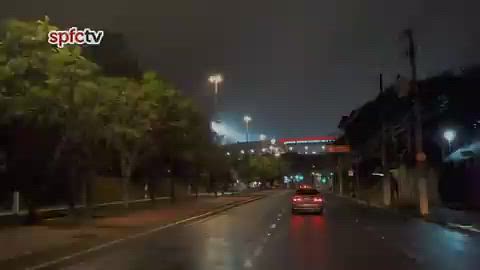The nighttime photograph captures a scene of traffic on a dark road illuminated by scattered streetlights. In the upper left corner, the image is marked with "SPFC TV." Predominantly, the line of cars occupies the middle lane, leaving the left and right lanes relatively clear. The taillights of the vehicles emanate a reddish-orange glow, enhancing the nocturnal ambiance.

On the right side of the road, several electrical poles stand tall, while a divider featuring green trees with brown trunks runs down the center. These trees might be planted in either pavement or dirt. Towards the foreground, the road seems to dip under a tunnel or an underpass, indicated by the structure ahead.

Green traffic lights hang above the scene, casting a subtle glow. Above these lights, there's a sign with red lettering, possibly belonging to a nearby sports arena. Additional streetlights are visible in the background, mingling with the night sky.

A road sign can be seen, though its details are indistinct. On the far right side, away from the divider, a figure might be walking, but it’s not clearly visible. The car in focus appears to be a sedan. The sky is a deep, dark black, setting a stark contrast with the artificially lit road below.